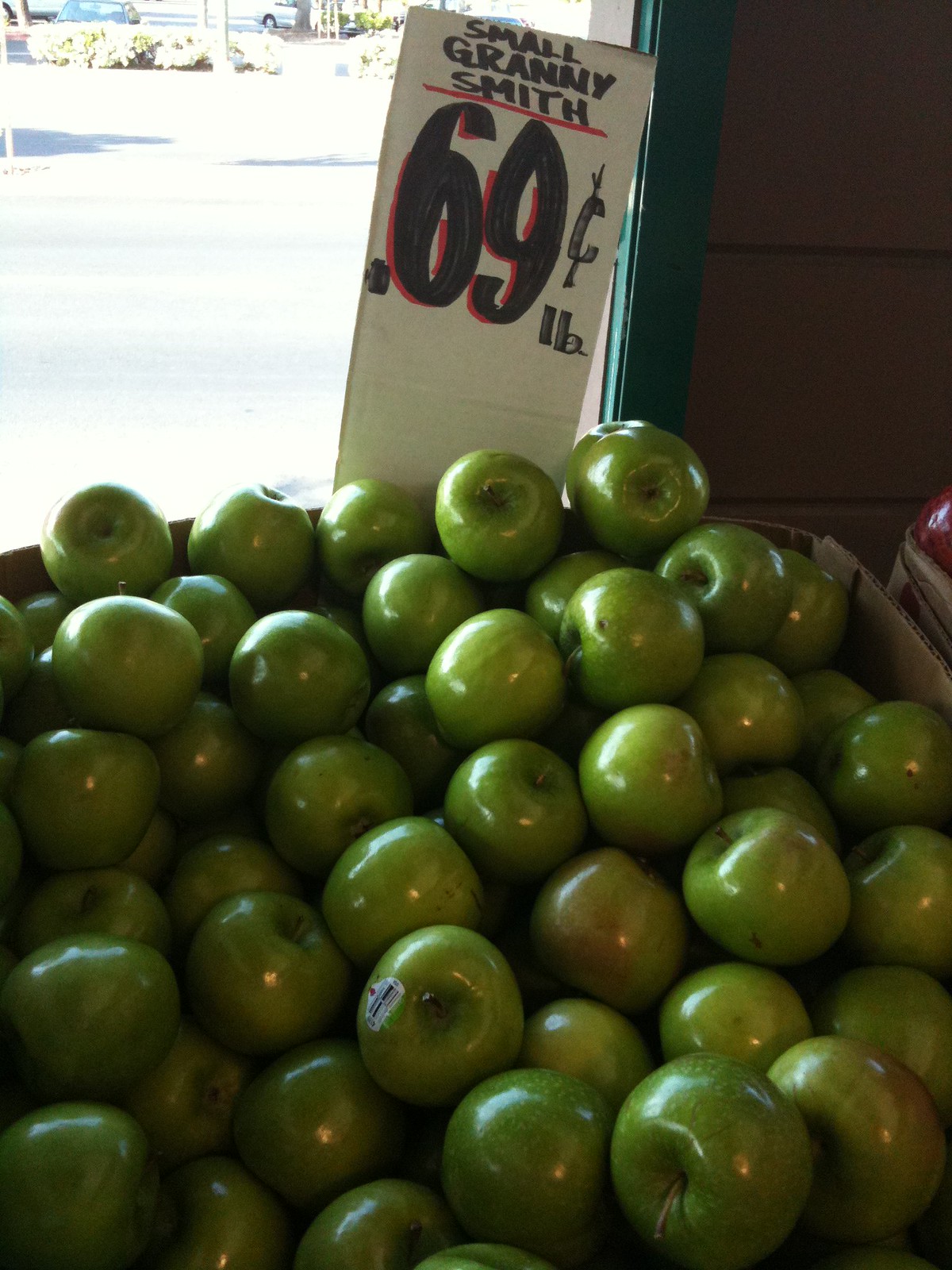In this vibrant image, we see a cardboard box brimming with small, glossy Granny Smith apples displayed at what seems to be a quaint produce market or corner store situated near a street. There are approximately 30 apples in view, each showcasing a vivid green hue, with some sporting a light touch of yellow and red, and a few adorned with identifying stickers. Behind the apples, a white cardboard sign, marked with handwritten text in magic marker, reads "Small Granny Smith, 69 cents a pound," underlined in red.

The setting is illuminated by bright sunshine pouring through a nearby window, casting a lively glow over the scene. Through the window, the street view reveals a broad sidewalk, a row of hedges, and a bustling road with parked cars. In the distance, poles and streetlights peek through, and the entire outside area appears to be blanketed in snow, adding a wintry charm to the otherwise vibrant display of apples.